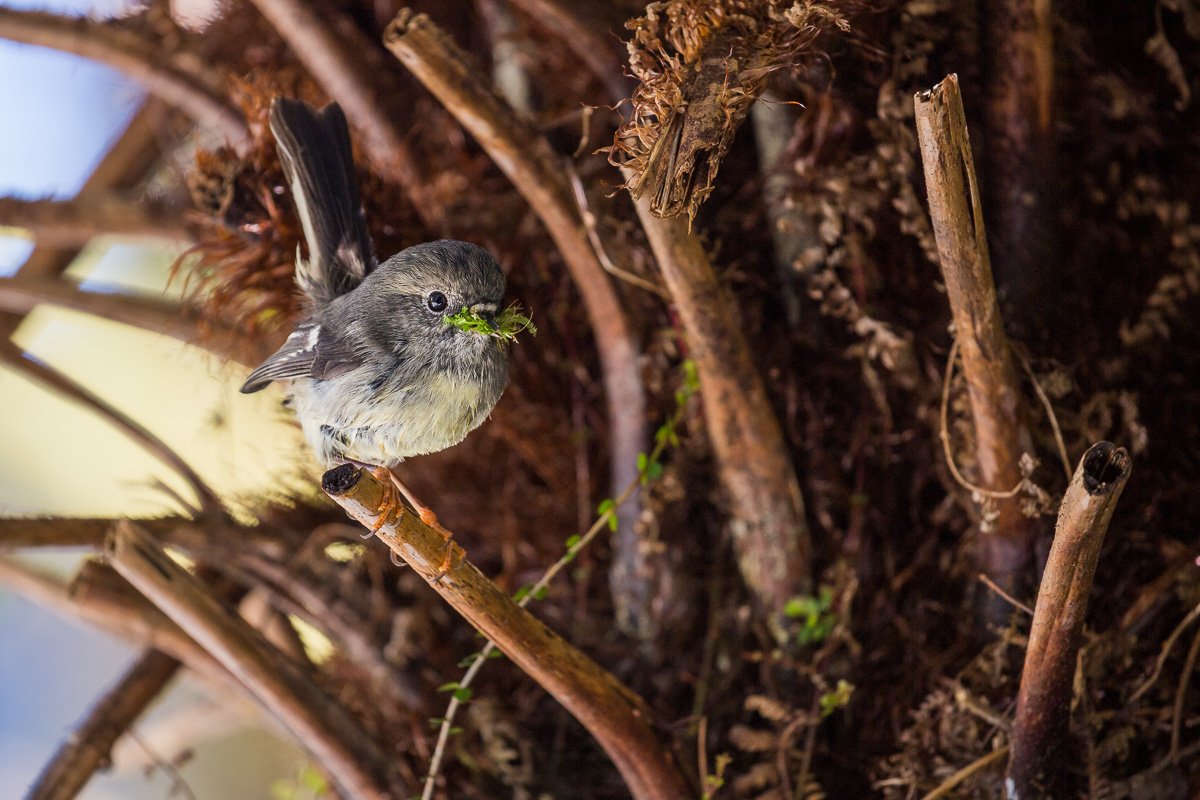The photograph captures a small robin perched on a branch jutting from a tree that predominantly occupies the right side of the image. The tree has numerous brown branches and protrusions that appear abruptly cut, surrounded by dead brown foliage and leaves. These branches extend across the image from right to left. The bird is positioned towards the left side of the image and is the main focus. It is perched with its small golden-colored talons on the branch, facing slightly to the right. The robin has a dark gray upper body with lighter gray feathers on its breast, and its tail feathers are also dark gray. It has dark black eyes and a gray beak, which is holding green leaves, possibly for nest-building. The background is mostly out of focus, highlighting the bird and branches, with a blue sky visible on the left side.